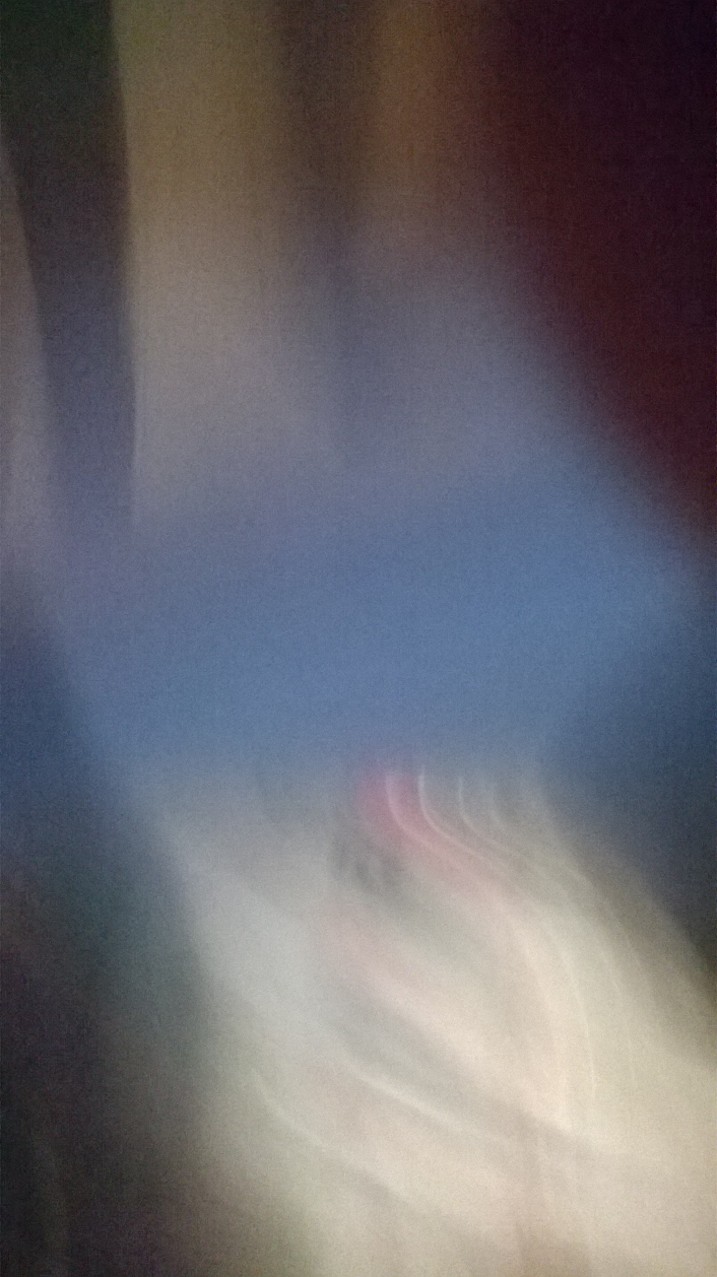The image is a completely blurred photograph that appears to have been captured with significant camera movement, making it largely illegible. It is vertically oriented, approximately twice as tall as it is wide. The sides of the image are very dark, almost black. In the middle, there is an irregular shape with a narrowed waist, featuring a mix of colors. At the top, a light blue area transitions into a white lower half, with streaks suggesting vertical camera movement. Additional details include a gray, bluish-gray bar extending from the upper left corner down into the center, and a horizontal, slightly tilted semi-rectangular area in the middle. There's a small pink or red spot at the center point, with several reddish wavy lines extending downward. The lower part of the image consists of white, cloud-like masses that resemble smoke or flames transitioning into smoke, with no distinguishable objects present.